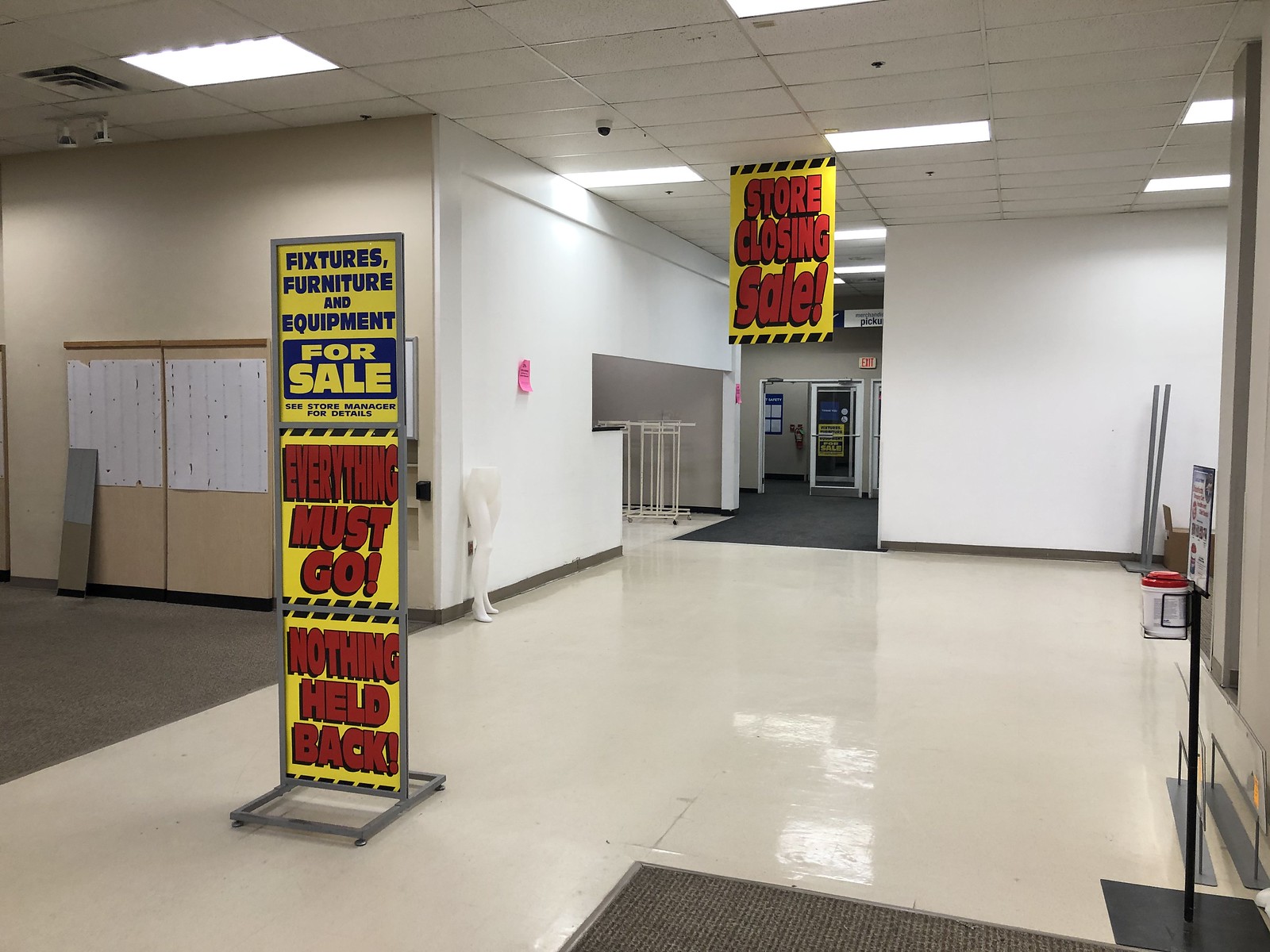The image displays the interior of an empty retail or furniture store that has gone out of business, marked by a sense of finality and abandonment. Dominating the top of the scene is a large banner declaring "STORE CLOSING SALE" in bold, uppercase red sans-serif letters against a yellow background. This sentiment is echoed across multiple signs that emphasize the urgency: "Fixtures, Furniture, and Equipment for Sale" in blue text on yellow, followed by "EVERYTHING MUST GO" and "Nothing Held Back" in red lettering. The space itself is stark and vacant, with tall white walls, interspersed with ceiling tiles and fluorescent lighting that accentuate the room’s emptiness. The floor is primarily green with commercial-grade gray carpet along the left side, while some remnants of white linoleum can be seen. The outdated ceiling panels suggest a structure that has withstood time but now stands desolate, showing no fixtures or furniture left, save for the prominent signs heralding its closure.